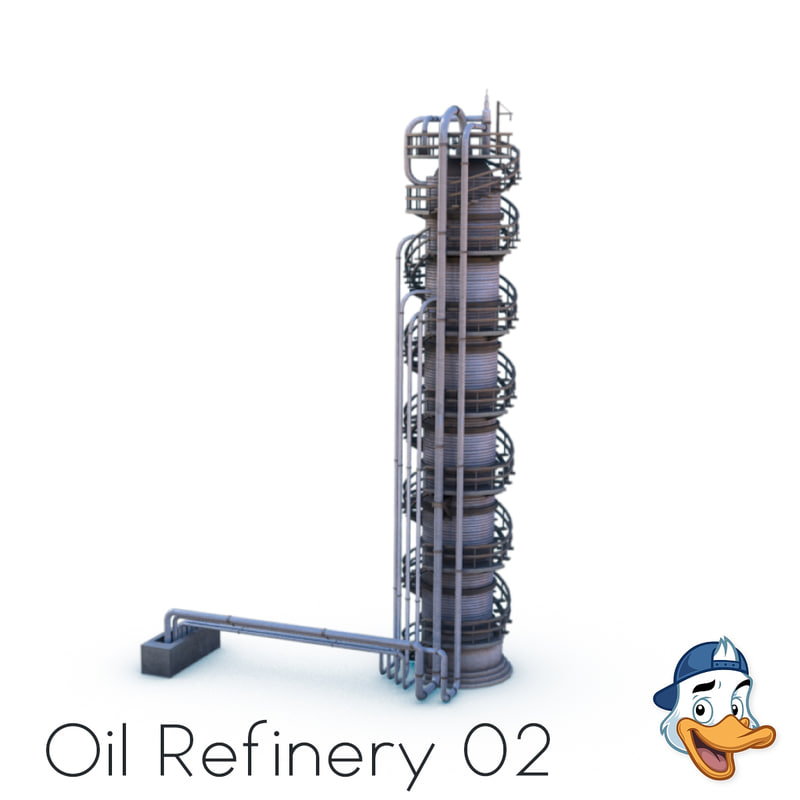The image showcases a computer-generated 3D model of a tall metal structure prominently positioned in the center against a fully white background. The structure features a cylindrical metal building encircled by a spiral staircase that ascends its entire height. Numerous metal pipes are attached horizontally and vertically, extending from a grey rectangular block. At the bottom of the image, in black text on a white background, it reads "Oil Refinery 02." To the lower right, there is an illustrated cartoon character of a duck with a white face, an orange beak, a happy expression, and a blue baseball cap worn backward with a tuft of hair peeking out. The duck appears to be smiling and looking to the left, adding a whimsical touch to the otherwise industrial setting. Shadows from the 3D model reflect subtly on the white ground, emphasizing the structure's detailed design.